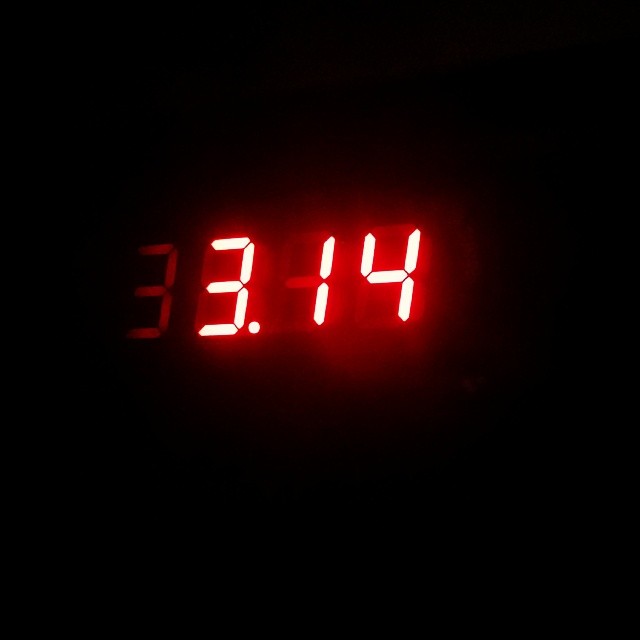This is an extreme close-up image of an illuminated digital display, likely from a device such as an alarm clock or a microwave. The screen is pitch black save for the bright, glowing digits "314" at its center. The display is framed by an unevenly lit backdrop, hinting at where other numbers or letters might appear if the setting or time were different. The rest of the image remains enveloped in darkness, providing no additional context or identifiable features of the device.